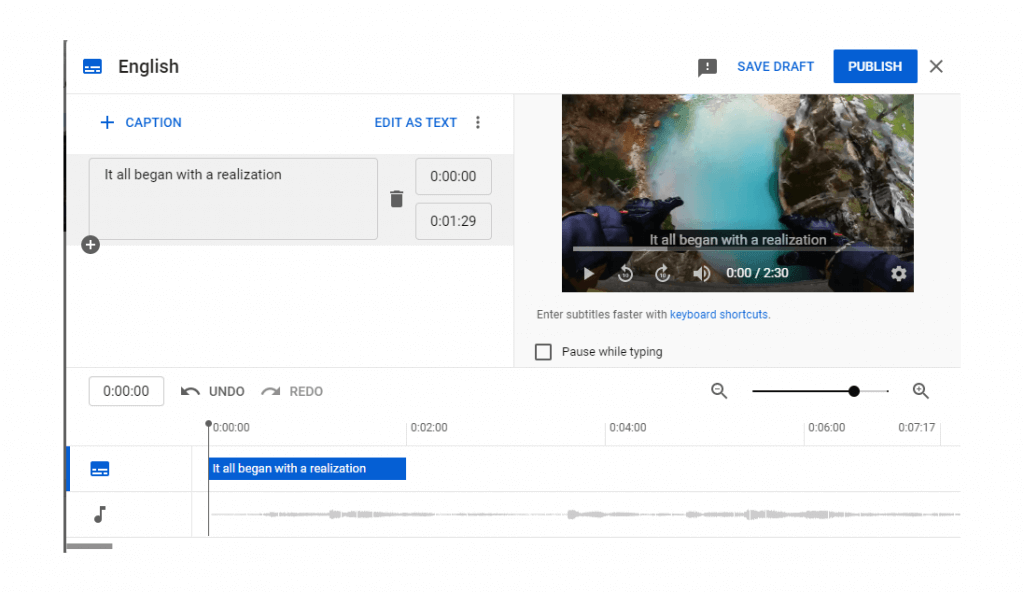This image showcases the interface of a likely web application designed for video or sound editing. The layout is horizontally aligned, making it suitable for tablets or desktop displays in portrait mode. The primary background color is white, complemented by black text and blue accents, which are predominantly used for interactive elements like buttons.

In the upper left corner, there's an option labeled "English" accompanied by a text symbol. At the bottom of the screen lies a light gray timeline, identified as a recording timeline by a black music note icon. A specific segment of the recording is flagged with the text, "It all began with a realization."

On the upper right corner of the interface, there's a paused video thumbnail featuring various video control options, including play, fast-forward 30 seconds, rewind 30 seconds, and a sound icon. The video duration is displayed as "0.00 seconds out of 2 minutes and 30 seconds," and a settings icon is present next to it. The thumbnail depicts someone diving into a blue pool, reminiscent of a scene from a video game, possibly resembling diving gameplay in "Call of Duty Warzone."

Overall, this detailed UI suggests a comprehensive video or sound editing application with diverse functionalities and an intuitive design.